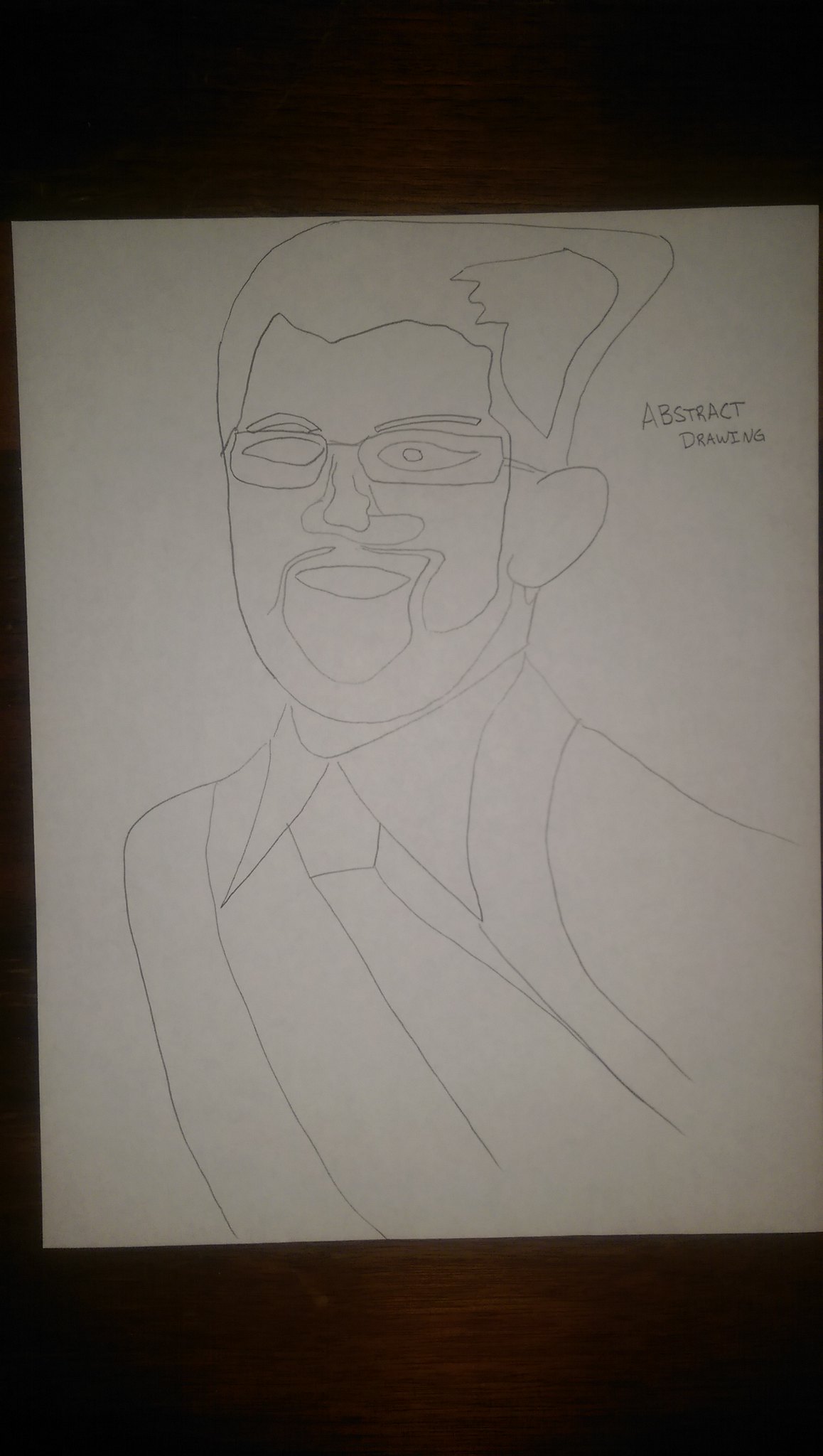The image is a photograph of a detailed pencil drawing on a white piece of paper, set against a dark wooden surface, likely part of a table. The drawing is of a man with a beard, wearing glasses, a suit coat, and a tie. The man's body is portrayed in a curved formation, and he is looking more towards the left side of the image. The drawing is stylistic, using outlines to define various features such as his long oblong-shaped eyes, the highlight in his hair, and details in his beard and nose. Additionally, there is text in the top right corner of the drawing that reads "ABSTRACT DRAWING" in capital letters, split over two lines.